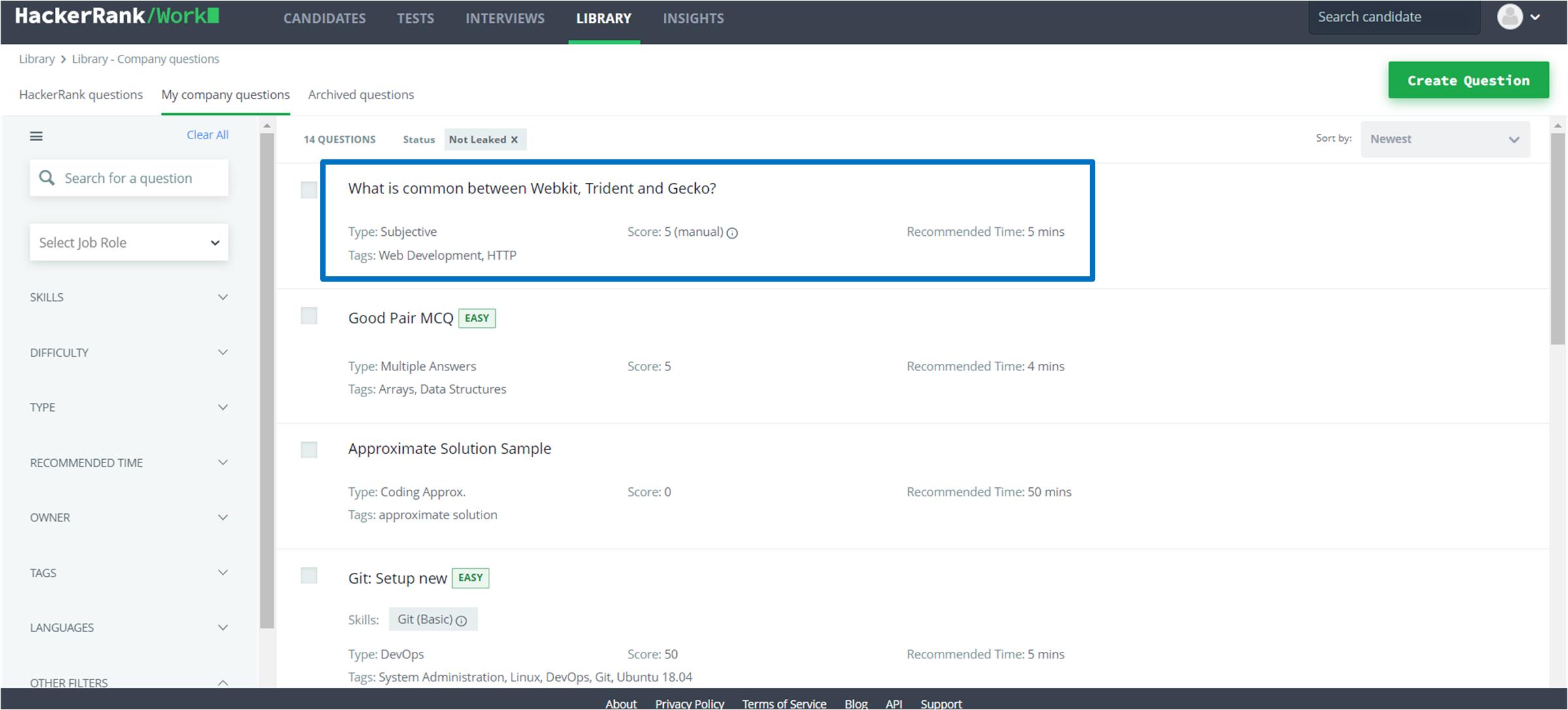This is a detailed screenshot of a HackerRank website interface viewed on a computer screen, likely a laptop or desktop. At the top of the image, there is a black navigation bar displaying several tabs: "Work," "Candidates," "Tests," "Interviews," "Library," and "Insights." The "Library" tab is highlighted in a brighter white, with a green underline indicating it is currently selected. On the right side of this bar, there is a search option labeled "Search Candidate" accompanied by an empty profile picture icon.

Just below the navigation bar, the interface continues with the header "Library" followed by a breadcrumb-like navigation path reading "Library > Company Questions." This is split into submenu options: "HackerRank Questions," "My Company Questions," and "Archived Questions," with "My Company Questions" being underlined in green, indicating it is the active selection.

Centrally positioned in the middle section of the screen, there is a list of questions. The first question is highlighted in a blue box, indicating it is the current focus. It reads: "What is common between WebKit, Trident, and Gecko?" This question is classified as "subjective" and tagged with "Web Development" and "HTTP." It carries a manual score of 5 points and has a recommended completion time of 5 minutes.

Below this is the second question titled "Good Pair MCQ," which is marked with a green "easy" label. It is a multiple-answer question, tagged with "Arrays" and "Data Structures," also carrying a score of 5 points with a recommended time of 4 minutes. Two additional questions appear listed beneath these, though are not fully detailed in the provided description.